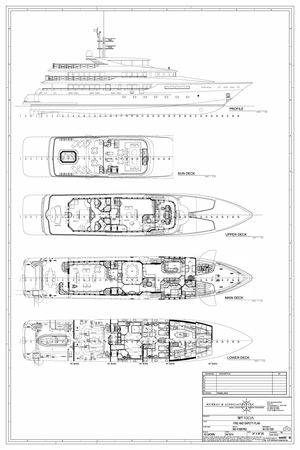The black and white poster-board image meticulously details the deck plans of a yacht, organized into five separate sections. The top portion provides a comprehensive side view of the entire yacht, showcasing its sleek design. Moving down, the second section illustrates the top deck, revealing seating arrangements, an open lookout area, and various rooms. The third section details the deck below, with additional seating, rooms, and a resemblance of a control room, possibly indicating its navigational functions. The fourth portion further explores another lower deck, meticulously highlighting different configurations, including identifiable areas like the galley and restaurant-like settings. Finally, the fifth and bottom section is the most intricate, presenting extensive rooms and facilities that occupy the lowest part of the yacht. Although minute, the diagram seems to include scaled measurements and a small, possibly certifying legend or certificate in the right corner, detailing the yacht's specifications and layout in a highly structured and informative manner, despite some unreadable text due to its blurriness.